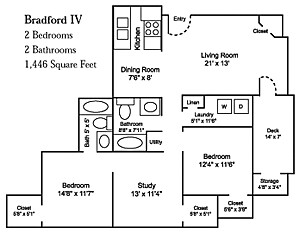This meticulously drawn, computer-generated floor plan of a Bradford IV apartment showcases a sophisticated black-and-white design. The caption underneath highlights its layout: two bedrooms, two bathrooms, encompassing a generous 1,446 square feet of living space.

The floor plan features an irregular shape rather than a standard square configuration. Entry is positioned at the top center, leading directly into the dining area and kitchen on the left-hand side. The kitchen is designed in a galley style, with the cooktop situated on the right side of the galley. The adjoining dining room measures 7 feet 6 inches by 8 feet.

Next to the dining room, the living room extends in an elongated form, spanning 21 feet by 13 feet. Two hallways emanate from the living space. One leads to an outdoor deck, which measures 14 feet by 7 feet. The other hallway guides you to a storage area, providing ample space for any belongings.

Proceeding down the second hallway, on the left, there is a bathroom equipped with a tub. Across from it, on the right, is a laundry room featuring a linen closet, complete with a washer and dryer for convenience. Further down, the utility closet is located on the right, followed by the entrance to the first bedroom, which measures 12 feet 4 inches by 11 feet 6 inches.

Continuing forward, the hallway leads to a study with an adjacent closet. Opposite the study, another bathroom is situated, also fitted with a tub. A closet protrudes from the left side, complementing the bedroom adjacent to it. This detailed layout ensures both aesthetic appeal and functional living in the Bradford IV apartment.